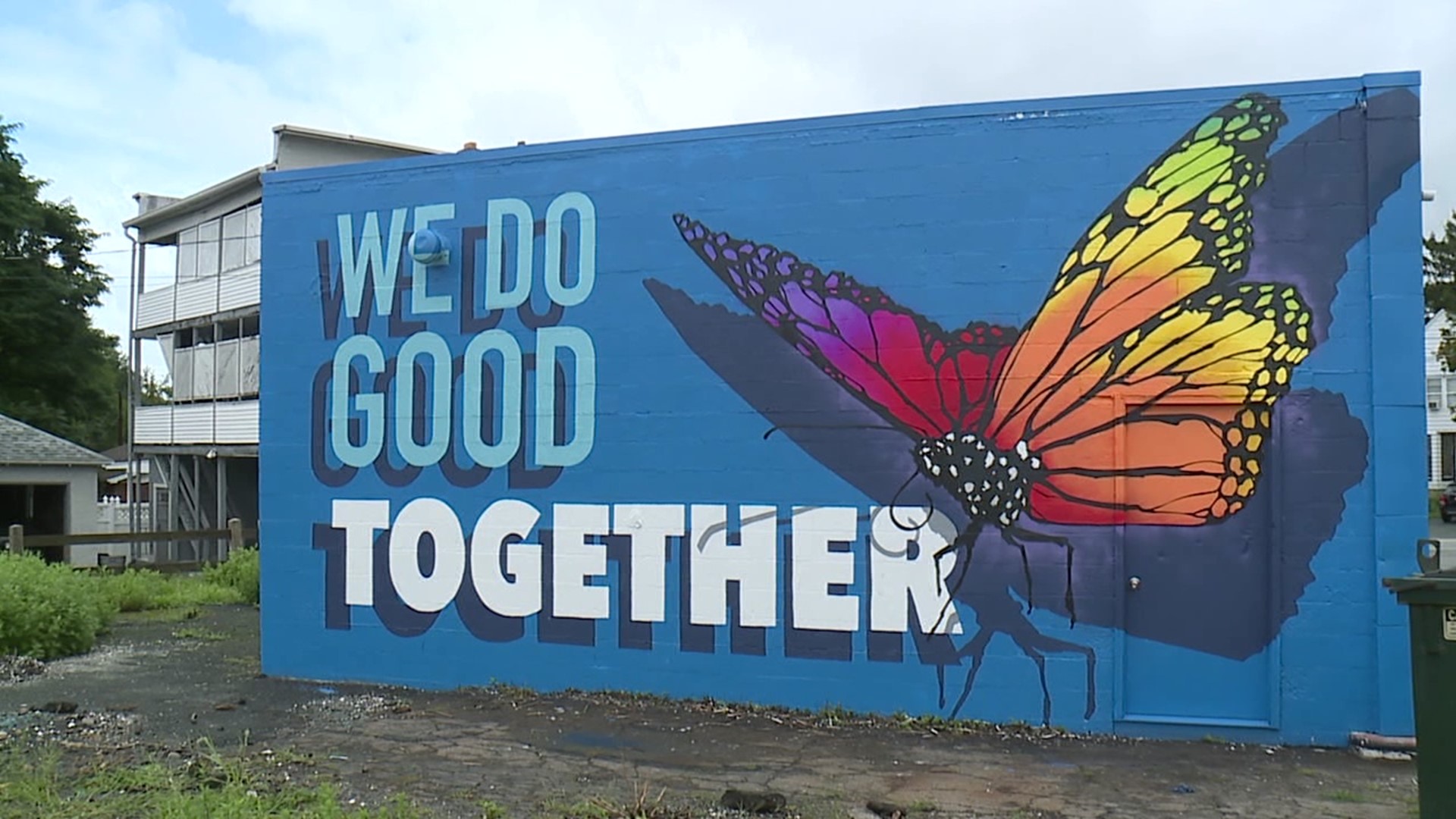This photo captures a vibrant mural painted on the side of a medium blue building. The mural features a light blue sky background with numerous clouds, making it appear expansive and airy. On the left side of the image, there's a white, two-story building with windows that appears taller and might be on stilts. Some greenery, such as green bushes and plants, is visible at the base of this building, adding natural elements to the scene.

The mural itself is the focal point, with a large image of a monarch butterfly. The butterfly's classic orange wings are accented with yellow at the tips, while its right wing transitions into shades of purple and reddish magenta. The entire butterfly is outlined in black and set against a dark grayish-purple backdrop, which provides striking contrast. To the left of the butterfly, light blue text reads "We do good," followed by thicker white text saying "Together," both with shadow highlights for added depth.

Within the mural, there is a doorway painted in blue that seamlessly blends into the artwork. The ground in front of the mural is a dark gray, muddy-looking path, and there's a section of concrete. Behind the mural, additional buildings are visible, including one with a slate or tiled roof, contributing to the layered architectural interest of the photo.